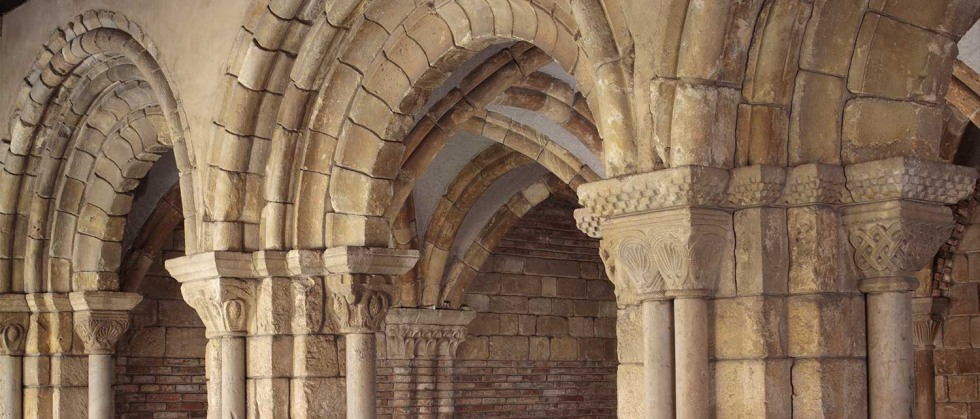The photograph captures a detailed section of an old, stone architectural building, showcasing its intricate design and craftsmanship. The focal point is an arrangement of two primary beige stone archways, flanked by a third partial arch that extends out of the frame. Each arch is adorned with various stone patterns and textures, leading to a series of columns halfway through the structure. Some of these columns exhibit distinctive carvings, reminiscent of Celtic rope designs. The image is cropped to emphasize the upper portion of the arches, revealing a background of brick-layered stone hallways that hint at the building's extensive, fortified architecture.